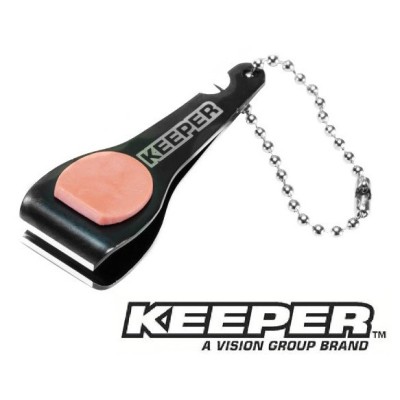The image displays a black nail clipper at a horizontal angle towards the left, prominently featuring a soft, oval-shaped padding on top that is a pinkish-peach color. The nail clipper bears the text "Keeper" in bold black lettering outlined in gray, followed by the phrase "Keeper, a Vision Group brand" beneath it. A silver chain is attached to the clipper, indicating it can be added to a keychain. The background is solid white, placing the nail clipper centrally in the frame, creating a clear and product-focused display apt for a sales advertisement.